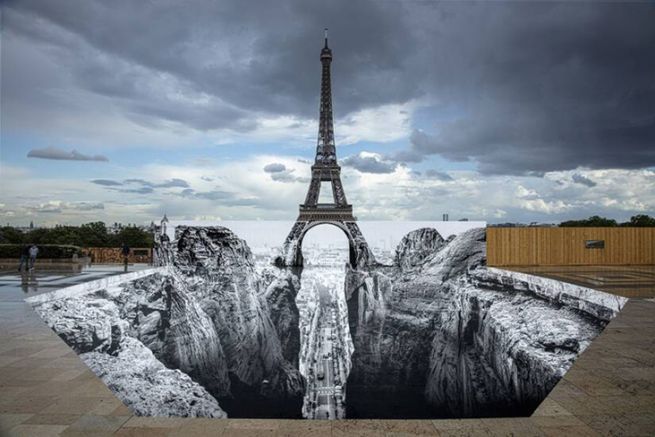In this surreal, computer-generated image, the Eiffel Tower has been placed in an extraordinary setting, spanning across a deep canyon with two opposite cliffs. Each of the tower's legs firmly stands on these grey and white cliff edges. Below the Tower lies a bustling city, with numerous cars navigating several roads, creating a stark contrast to the Tower's isolated placement. The sky above is a turbulent mix of dark grey clouds, sporadic patches of blue, and some white clouds near the horizon line. Towards the background, beyond the Eiffel Tower, there appears to be a pool or a frozen body of water, casting a white reflection and adding to the image's ethereal quality. The bottom arch of the Eiffel Tower allows for a downward view through to this reflective surface. On either side of the image, a wooden deck with a brown wooden fence frames the scene, grounding the otherwise fantastical landscape.